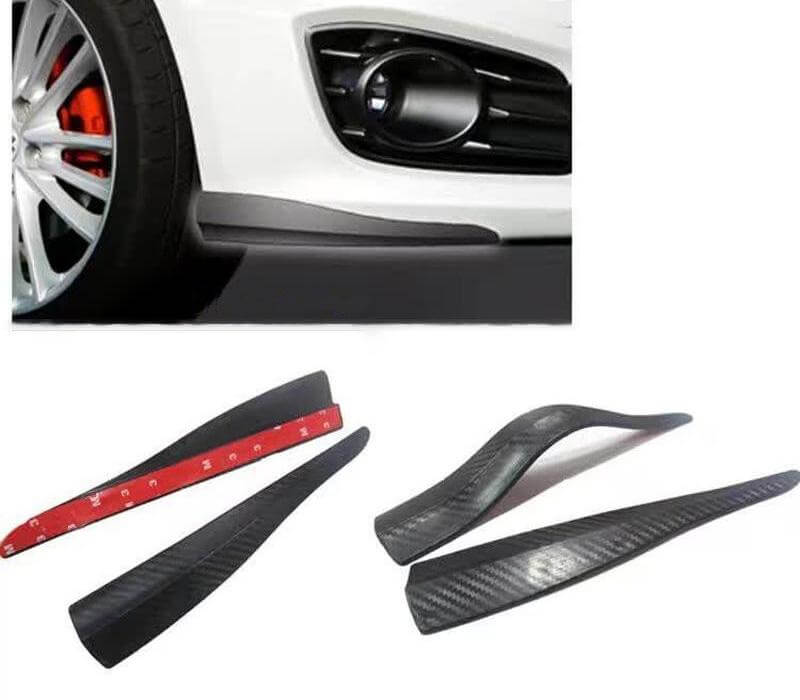The image depicts a detailed product photo for a sleek car accessory designed for the front bumper. At the top, there is a photo of the bottom front corner of a white car's bumper, showcasing the mounted lip accessory with a subtle white gradient highlighting its placement. The car features a black tire with a stainless steel rim, partially visible with an orange element underneath. Below the car image, the accessory itself is showcased in two smaller images. The left image exhibits two strips of carbon fiber with alternating dark and light gray stripes, indicating flexibility with 3M double-sided red adhesive tape on the back. The right image shows one strip with a curved shape and another in a flat position on a white surface, further emphasizing their adaptable design. The accessory is universally applicable, enhancing the sporty aesthetic of the car.